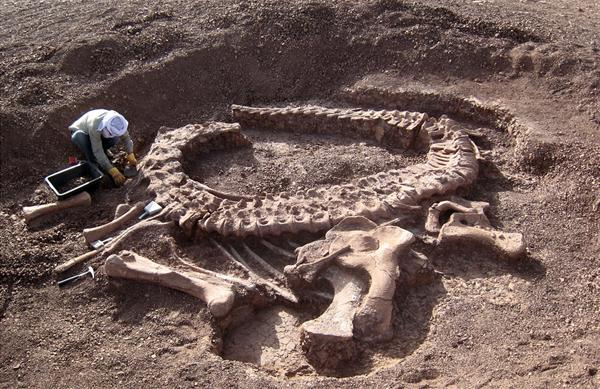In this detailed outdoor scene, a person is kneeling in a dirt pit, excavating a large set of dinosaur bones. The soil appears in muted tones of burgundy brown and grayish brown, complementing the dull hues of the fossils. Central to the image is an enormous, fossilized tail coiled in a circular formation, its sheer size dominating the composition. The tail's segments are so vast that they create areas of dirt within the coils. Alongside the coiled tail, various other colossal bones are scattered around, including what appear to be leg and shoulder bones, some of which are larger than the person.

Positioned on the left side of the image, the individual wears blue jeans, a gray shirt, tan gloves, and a white head covering, likely for sun protection. Beside them lies a small black container or box, presumably for collecting artifacts. The scene vividly portrays the meticulous work of excavation amid the grandeur of prehistoric remains.